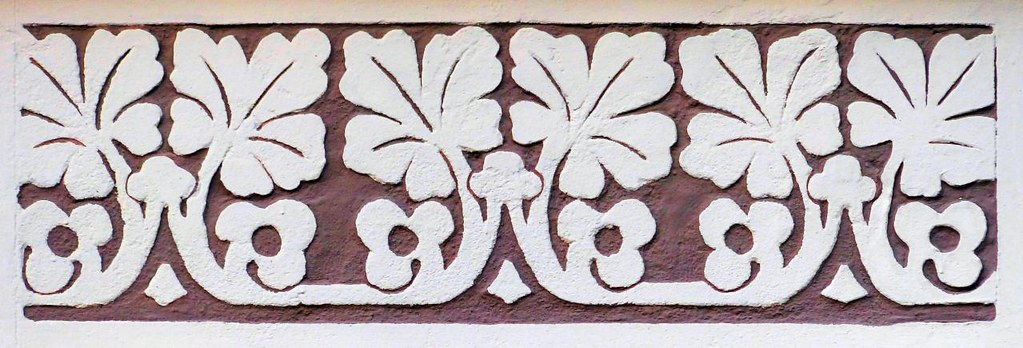This image showcases a decorative concrete panel with a sophisticated design that merges artistic and floral elements. The panel features a dual-color scheme with a gray base, burgundy or brown recesses, and white extruded elements. The trim is entirely white and borders the panel elegantly.

In the center, there are three identical symmetrical patterns. Each pattern consists of floral shapes that resemble two large five-leaf clovers or flowers fanning outwards with their petals blossoming. The middle of this floral design features a club-like shape, similar to the clubs in a deck of playing cards, flanked by larger clubs with circles at their centers. At the bottom of each floral pattern, a white bell-shaped design completes the intricate and symmetrical motif. This panel is likely designed to be a decorative installation on a wall, combining artistic detail with precise symmetrical patterning.